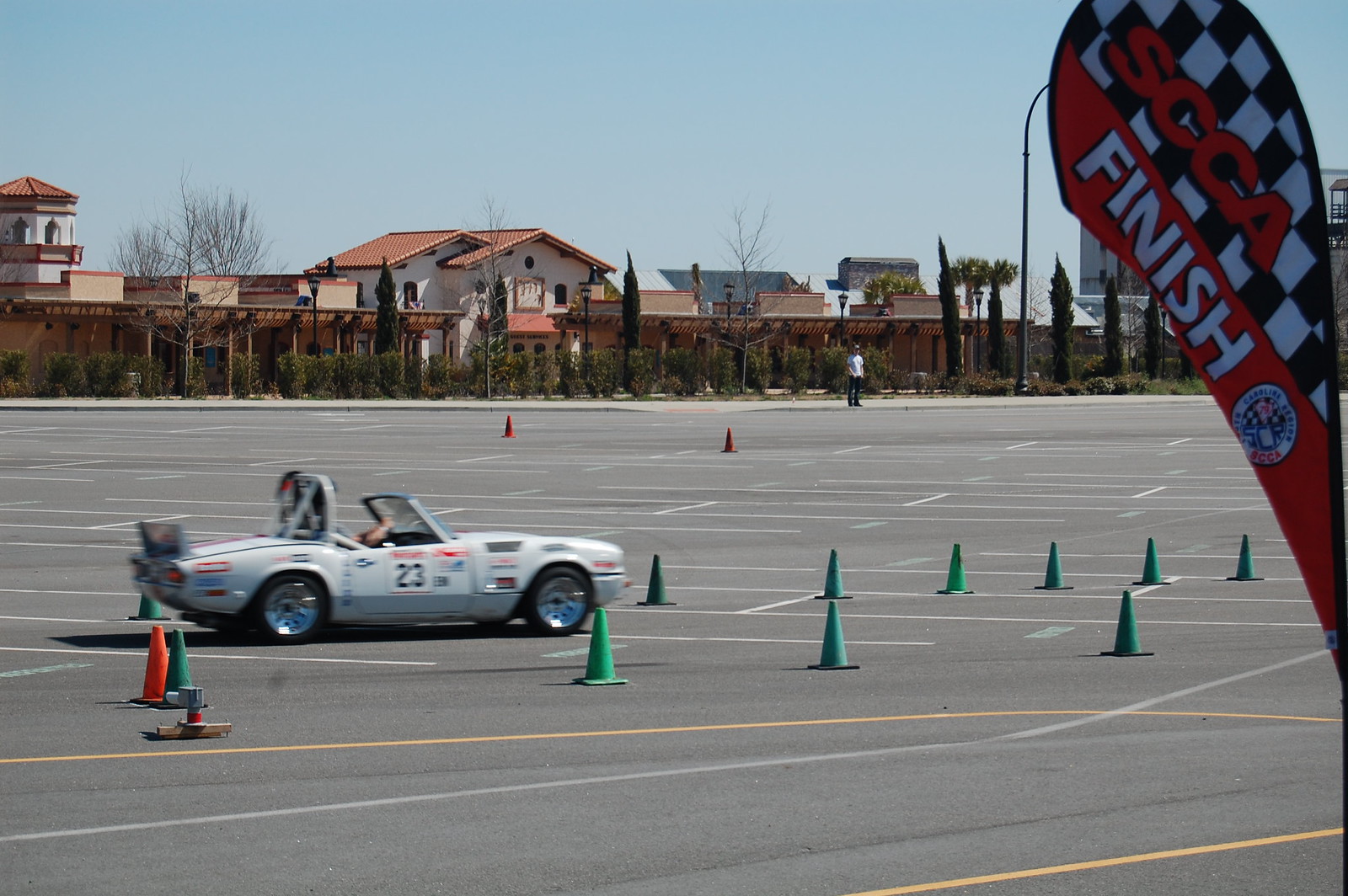The image captures a light gray sports car with the number 23 painted on its right door, situated in a vast parking lot filled with various colored traffic cones, predominantly green, with a few orange and blue ones scattered around. The car appears to be a convertible with its roof down, driven by a single occupant. The parking lot is relatively empty, with the notable presence of a finish banner that reads "SCCA Finish" in the upper right corner, indicating a possible involvement in an automotive event. There is a mix of pavement markings, including white and yellow stripes, and a person can be seen standing at the far end of the parking lot. The background features a sidewalk, bushes, small trees, and buildings under a clear blue sky. The image is slightly blurry around the car, suggesting it may be in motion.